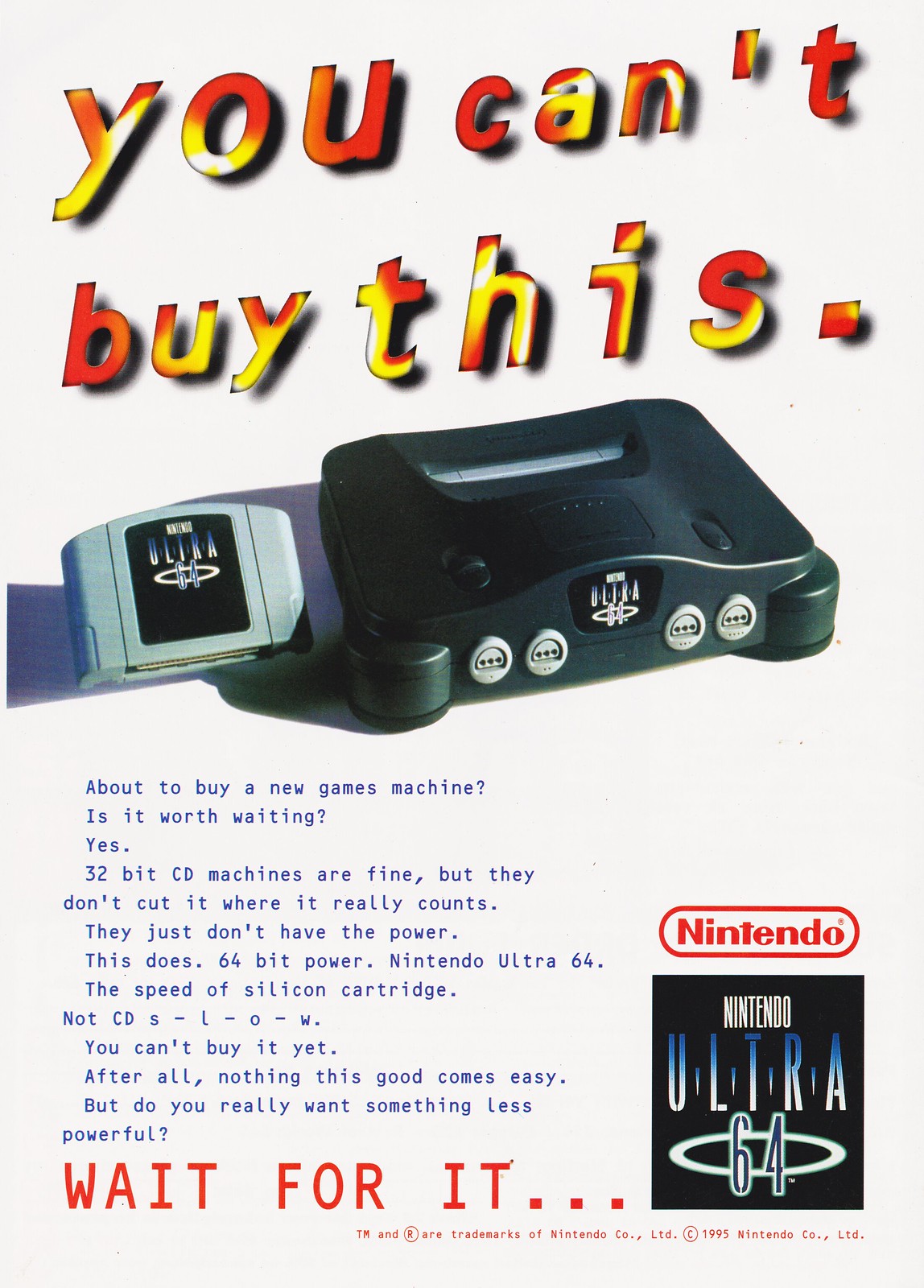This tall, rectangular advertisement features a light gray background. Dominating the top, tilted upwards with an energetic vibe from the 90s, is a vibrant and eye-catching text that voraciously declares, "You can't buy this. Period." This statement is illustrated in a striking blend of bright red, yellow, and white colors, with each letter casting a realistic shadow, adding depth and a hovering effect. Below this bold proclamation, a small black game console is showcased alongside a gray game cartridge labeled "Ultra 64."

Further down, the advertisement addresses potential buyers with small, blue, detailed text posed like a conversation starter: 

- Are you about to buy a new games machine? Is it worth waiting?
- Yes.
- 32-bit CD machines are fine, but they don't cut it where it counts. They just don't have the power. This does. 64-bit power. Nintendo Ultra 64.
- The speed of a silicon cartridge, not CD-S-L-O-W.
- You can't buy it yet. After all, nothing this good comes easy.
- But do you really want something less powerful? Wait for it...

The information is capped off with a final line in prominent red block lettering: "Wait for it..." In the lower right-hand corner, the familiar red Nintendo logo also sits next to a small black emblem reading "Ultra 64" in white text, encircled with a ring in the background. This detailed advertisement feels like a snapshot from a 90s magazine, promoting what would become an iconic era for Nintendo.